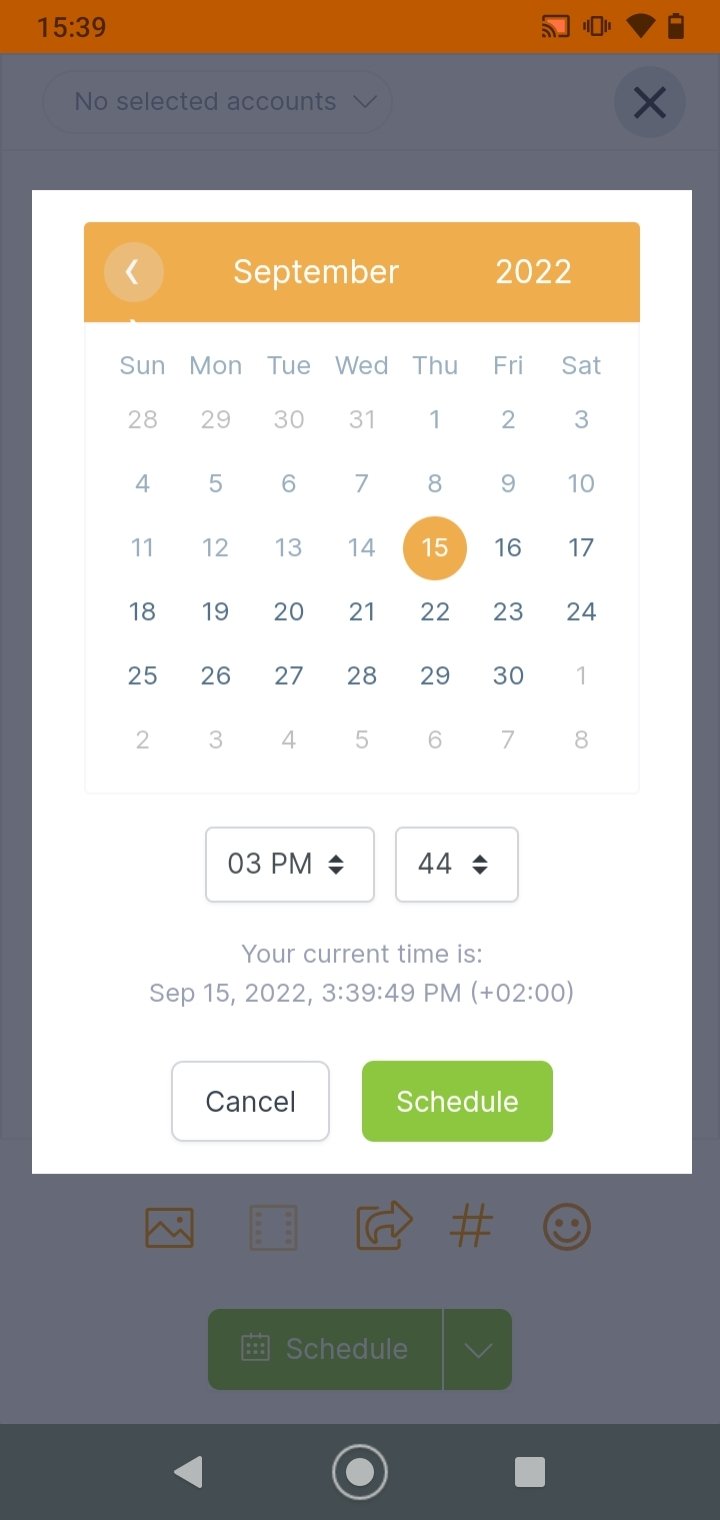A screenshot of a smartphone display shows a detailed view of the calendar interface under the "Schedule" menu. The calendar, set to September 2022, is positioned prominently in the middle, with all the dates displayed in gray. The past dates are distinguished by a lighter gray hue. At the bottom of the calendar interface, there's a dropdown menu to select specific times, accompanied by a display of the current time. Two buttons are present beneath the calendar: a white "Cancel" button and a green "Schedule" button. The background of the interface is grayed out, indicating the user has clicked on the "Schedule" option. At the top of the screen, an orange status bar displays the time in military format (15:39), along with icons indicating the battery level and Wi-Fi connectivity.